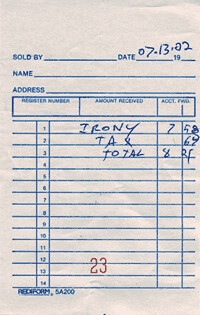This image displays an old-fashioned paper receipt, slightly off-white in color with a touch of gray and handwritten in blue ink. The receipt, appearing as if it's from a pad with carbon copies, is sparsely filled out. At the top, there are fields for "Sold by" and "Date" – the latter filled out with "07-13-02" or "07.13.22". Below this, blank lines await the "Name" and "Address". Further down, there are fields labeled "Requester Number", "Amount Received", and "Account Forward", all empty. Sequentially numbered lines from 1 through 14 are present, with detail on the first line indicating an item described as "irony" priced at $7.58. The tax listed is $0.69 or $0.64, though this discrepancy makes the total ambiguous, but noted as $8.21. Notably, a red number "23" appears between lines 12 and 13.